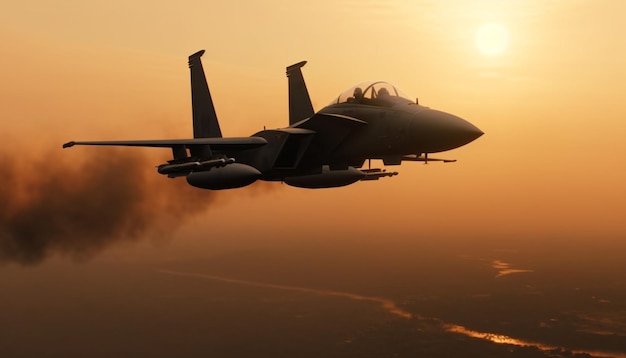In this fully-aligned rectangular image, a dark gray fighter jet with two vertical tailfins is captured in mid-flight, viewed as if from an adjacent plane. The jet, which features a pointed nose and carries two pilots beneath a domed canopy, emits a dark brown or black stream of smoke from its rear. The sky around the jet is tinged with a red-orange hue, appearing foggy and smoggy, causing the sunlight—depicted as a slightly obscured, small yellow circle in the upper right corner—to appear faint. Below, the land transitions from dark tan at the horizon to darker brown or gray near the bottom, where a narrow body of water runs diagonally from the lower right to the left side of the image, suggesting the jet is flying over a valley.